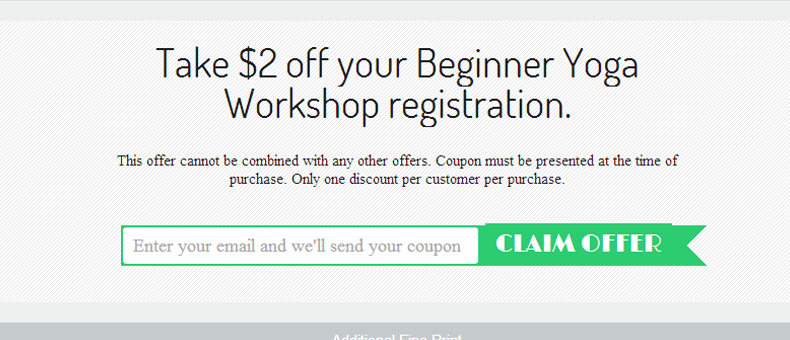Screenshot of a promotional website banner with detailed design elements:
The banner features a grey background with a prominent, bold black title stating, "Take $2 Off Your Beginner Yoga Workshop Registration." Below the title, there is smaller black text detailing the offer: "This offer cannot be combined with any other offers. Coupons must be presented at the time of purchase. Only one discount per customer per purchase." Below the main promotional message, there is a grey banner with additional fine print in white text, although partially cut off. On the right side, there is an interactive section featuring an email input bar, which has a green outline and a white interior, and a green "Claim Offer" button with "Claim Offer" written in bold white block letters.